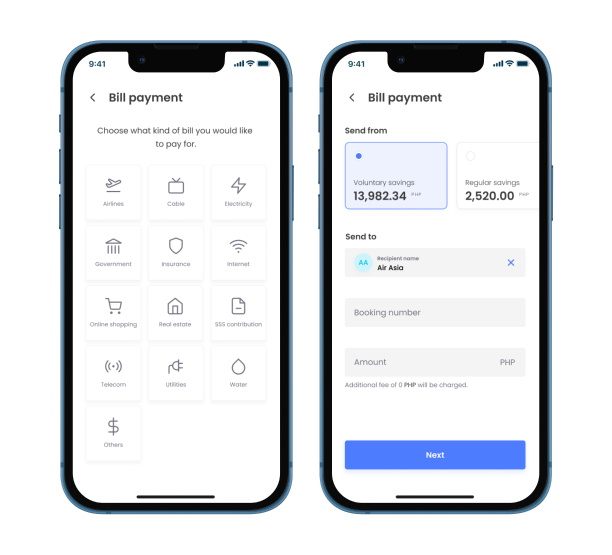In this image, we observe two smartphones placed side-by-side against a pristine white background, showcasing screenshots of their respective screens. Each smartphone features a sleek black frame that sharply contrasts with the bright backdrop.

On the left screen, we see a bill payment interface. The top of the screen displays the standard status icons: the time set at 9:41, a fully charged battery indicator, alongside icons for signal strength and wireless connectivity. Just beneath these icons, the text "Bill Payment" stands prominently. Following this, the prompt "Choose what kind of bill you would like to pay for" guides the user through the process. The interface is neatly arranged into four rows, with three icons per row, each representing different bill categories. For example, the first row includes:
- **Airlines**: Illustrated by a simplistic plane icon.
- **Cable**: Represented by a basic TV drawing.
- **Electricity**: Depicted with a straightforward lightning bolt symbol.

The right screen continues the bill payment process, mirroring the same status icons at the top and time set at 9:41. The heading "Bill Payment" is still present, indicating the continuation of the task. Below, the interface advances to the step where the user specifies the payment details. It starts with "Send from," presenting two options:
- **Voluntary Savings**: Showing a balance of $13,982.34.
- **Regular Savings**: Showing a balance of $2,520.00.

Underneath this section, the "Send to" part confirms the chosen recipient, which in this case is AirAsia. The bottom of the screen includes a prominent blue button labeled "Next" in white text, providing a clear call-to-action for proceeding to the next step. 

Overall, the clean and detailed design clearly guides the user through the bill payment process on both interfaces.